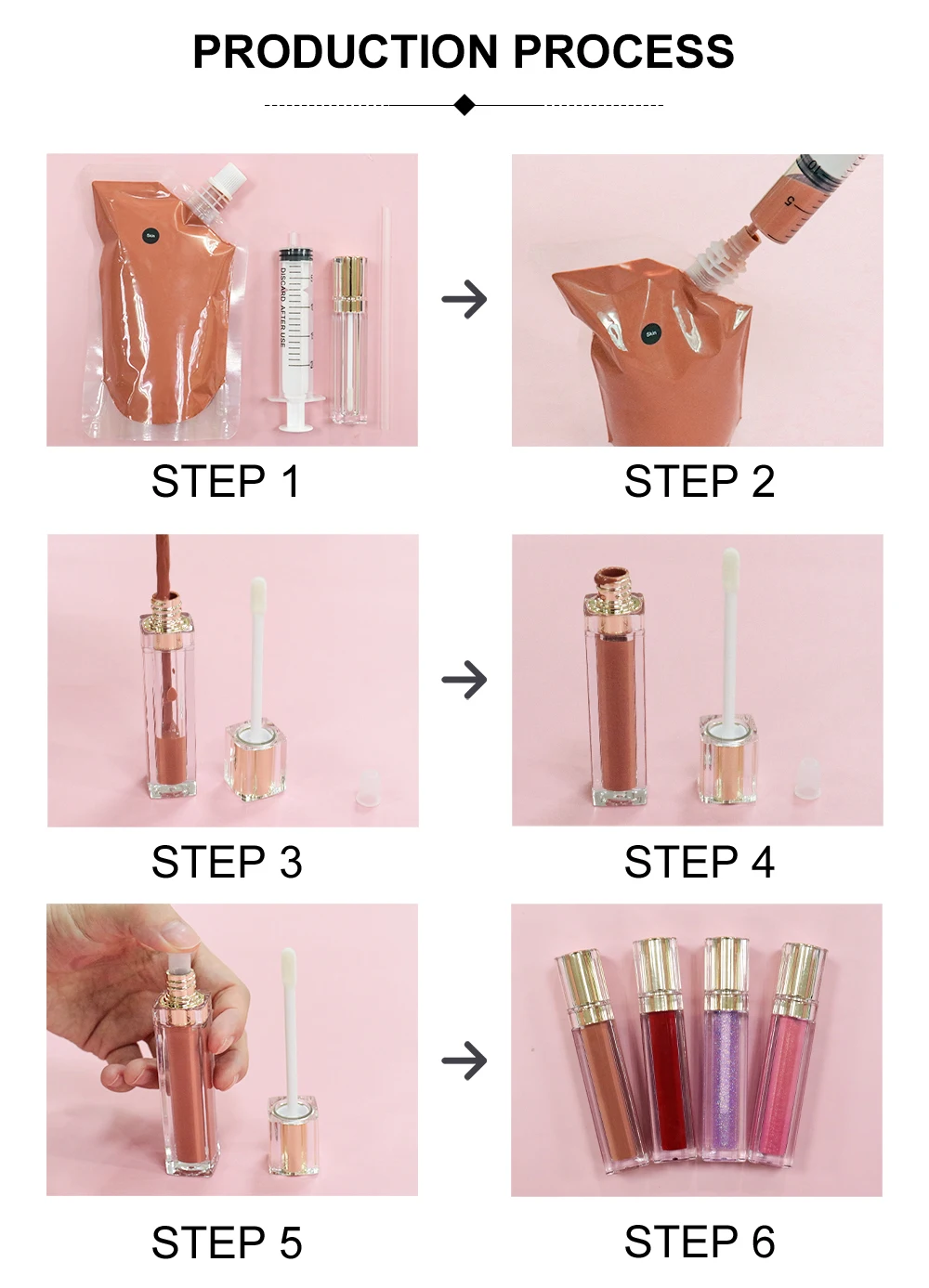This detailed illustration shows a step-by-step production process prominently titled in bold uppercase black font across the top on a white background. Below, there are six smaller rectangular images arranged in two vertical rows against a pink backdrop, each capturing a different step, numbered from Step 1 to Step 6, with black diamond shapes and arrows indicating the flow. 

In Step 1, a tan plastic pouch with a tube and cap meets three objects to the right, including a syringe and possible testing strips or a clear empty bottle with a gold cap. Step 2 depicts the syringe extracting brown liquid from the pouch. Step 3 shows the syringe positioned to fill a tube partially, a stream of liquid descending into it. In Step 4, a gloss tube stands filled with a sponge applicator next to it. Step 5 captures a hand inserting the applicator into the tube, emphasizing attentiveness to detail. Concluding in Step 6, four colored tubes, likely gloss or nail polish, are neatly aligned side by side, showcasing the final product ready for use. This flowchart uses photographic realism to clearly delineate the stages of producing liquid lip gloss or a similar cosmetic item.